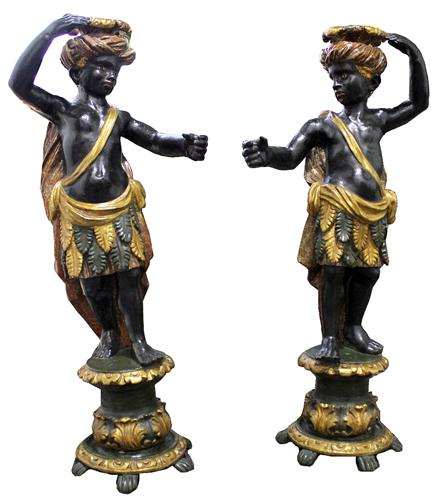The image showcases two statues that appear to be mirror images of each other, featuring a high level of detail and craftsmanship. Both statues depict young, black-skinned characters adorned with a gold sash draped across their chests and a skirt displaying an intricate pattern of alternating bronze or gold and black leaves. The figures stand on heavily detailed cylindrical pedestals, which share the same bronze and black coloration as their attire. Each statue has one arm extended outward as if holding a cup, while the other arm reaches toward the top of their head. Atop their heads, they wear black and gold turbans, which are further topped by what looks like a bowl or plate, perhaps suggesting their use as candlestick holders. The overall appearance suggests ancient or historical art, lacking any background or borders to contextualize the scene further.